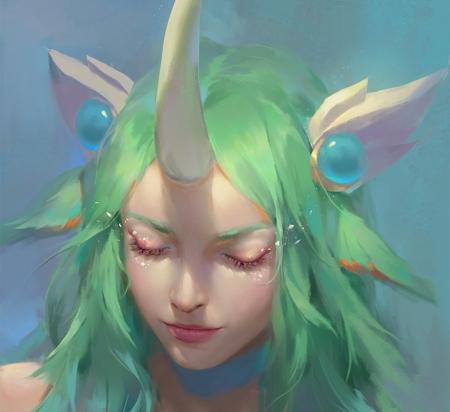This image portrays a fantastical, ethereal young woman rendered in a dreamy, watercolor style with a predominantly light blue, textured, pastel background. The character, appearing to be in her early 20s with very light skin and of European descent, has vibrant green hair with feather-like textures and subtle orange streaks around the front of her head. Her eyes are closed, highlighted by glitter on her eyelids, giving her a serene, otherworldly demeanor. 

She features striking green eyebrows and light pink lips, accompanied by a large, spiraling white horn protruding from the center of her forehead. Adorning her head are what seem like animalistic ears, doubled up – large ones flaring out and a second green pair beneath them. Each ear or wing-like appendage is embellished with blue glass ball-like pearls. Around her neck, she wears a delicate blue ribbon. Overall, the piece has a glowing, aura-like quality, immersing the viewer in a fantastical, dreamlike atmosphere.